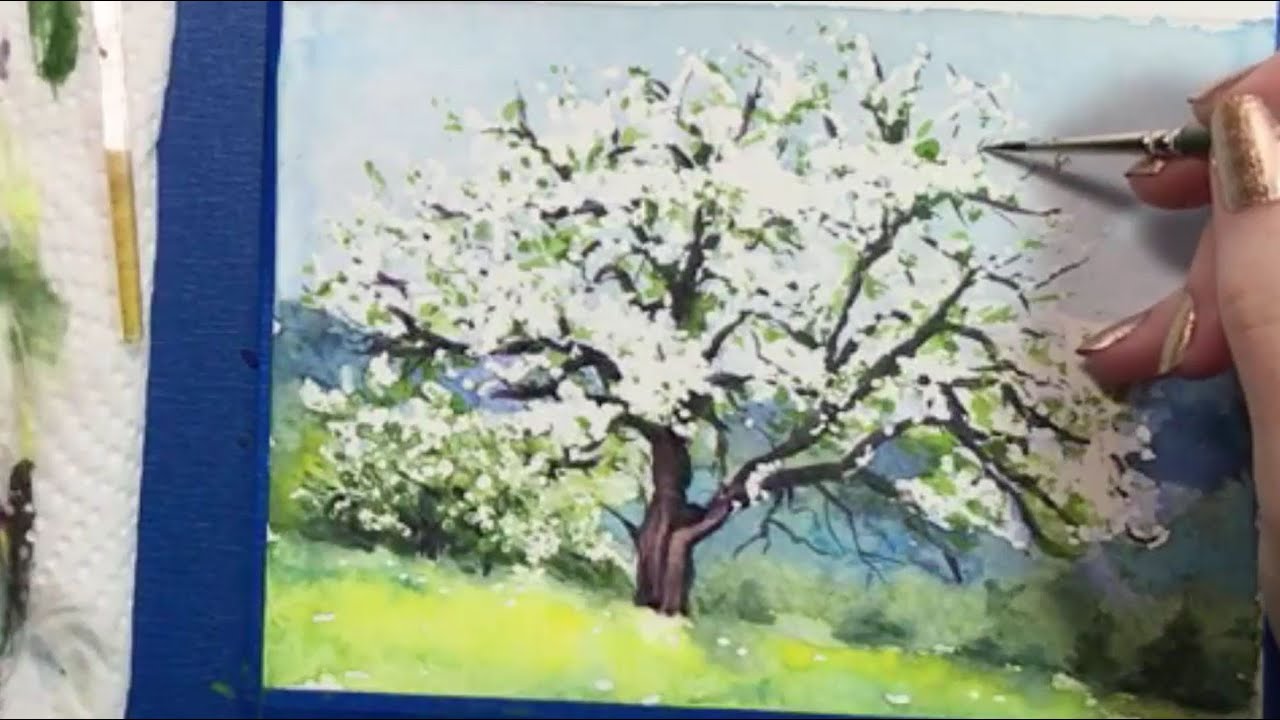This photograph captures a detailed scene of a female artist, identifiable by her Caucasian skin and gold-painted fingernails, intricately painting a blooming tree. The artist's fingers, partially seen on the right side of the image, hold a fine-tipped paintbrush, suggesting she's applying detailed strokes. The tree, which appears to be in full bloom with numerous white flowers and sparse green leaves, stands out against a backdrop of vibrant green grass and surrounding shrubbery. The tree's dark brown, short trunk supports a dense, bushy network of thick branches. Above, the sky is a clear blue with minimal clouds, adding depth to the scene. The composition hints at other elements such as a piece of paper towel with green and yellow smudges, possibly from previous brush cleaning, and some blue tape framing the canvas. The artist's workspace suggests a blend of oil and watercolor techniques, contributing to a somewhat Impressionist style that captures the essence of a wild-shaped fruit tree in a picturesque meadow.